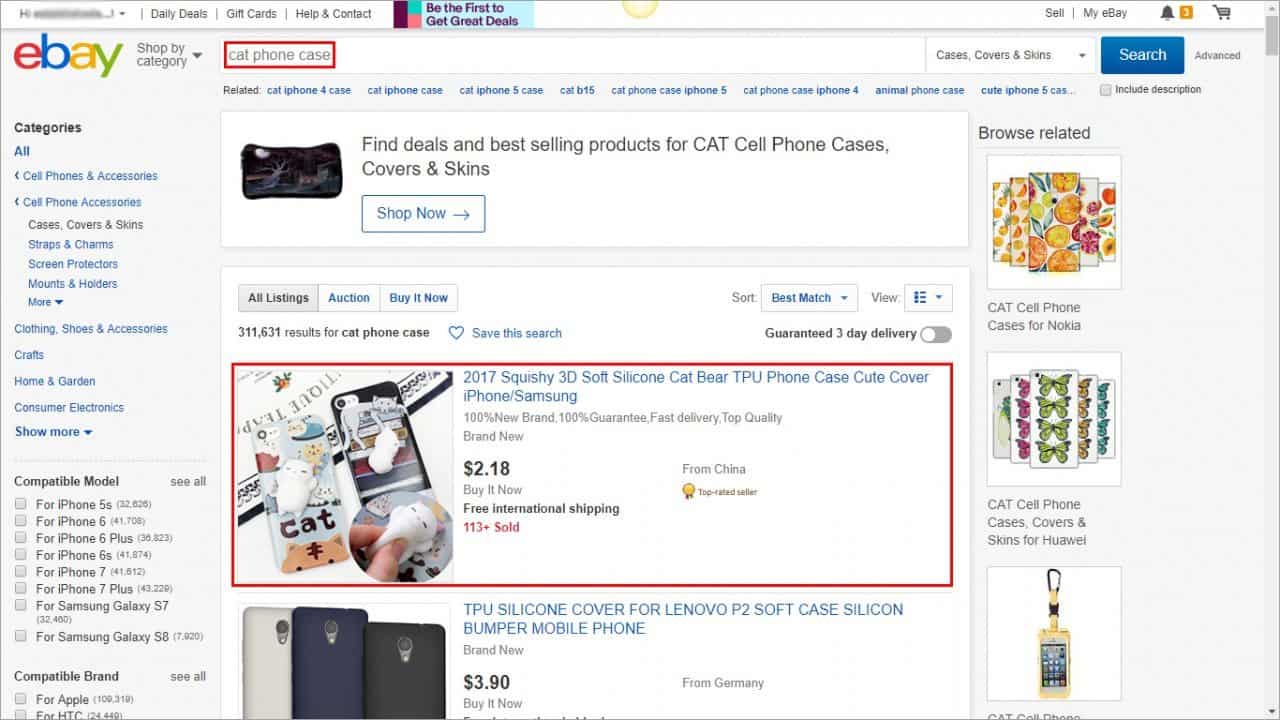A detailed screenshot of an eBay webpage is displayed. In the upper left corner, partially obscured by digital scratching, it shows "Hi" followed by the site's basic navigation links: "Daily Deals," "Gift Cards," "Help & Contact," and the motivational message "You're the first to get great deals." On the right-hand side, the options "Sell," "My eBay," an icon of a bell (possibly for notifications), and a shopping cart are visible. The iconic multicolored eBay logo is prominently featured in red, blue, yellow, and green next to the phrase "Shop by category."

Standing out in red is the search term "cat phone case." Below this, on the left sidebar, highlighted in white, is the “Categories” section. Listed under it, in blue text, are options including "Cell Phone Accessories," leading to subsections like "Cases," "Color Skin," "Straps," "Charms," among other phone-related items, indicative of a focus area for mobile accessories.

The listings suggest this is an older screenshot. The devices referenced, such as the iPhone 5S and Samsung Galaxy S7, S8, align with product offerings around 2017. Featured prominently is a "2017 Squishy 3D Soft Silicone Cat Bear TPU Phone Case," noted as "cute" and suitable for various iPhone and Samsung models, accentuated with a black border. Another listing at the bottom showcases phone cases in gray, blue, and black, designed for a device with a large, centrally-placed camera, implying a specific, older smartphone make and model suitable for these cases.